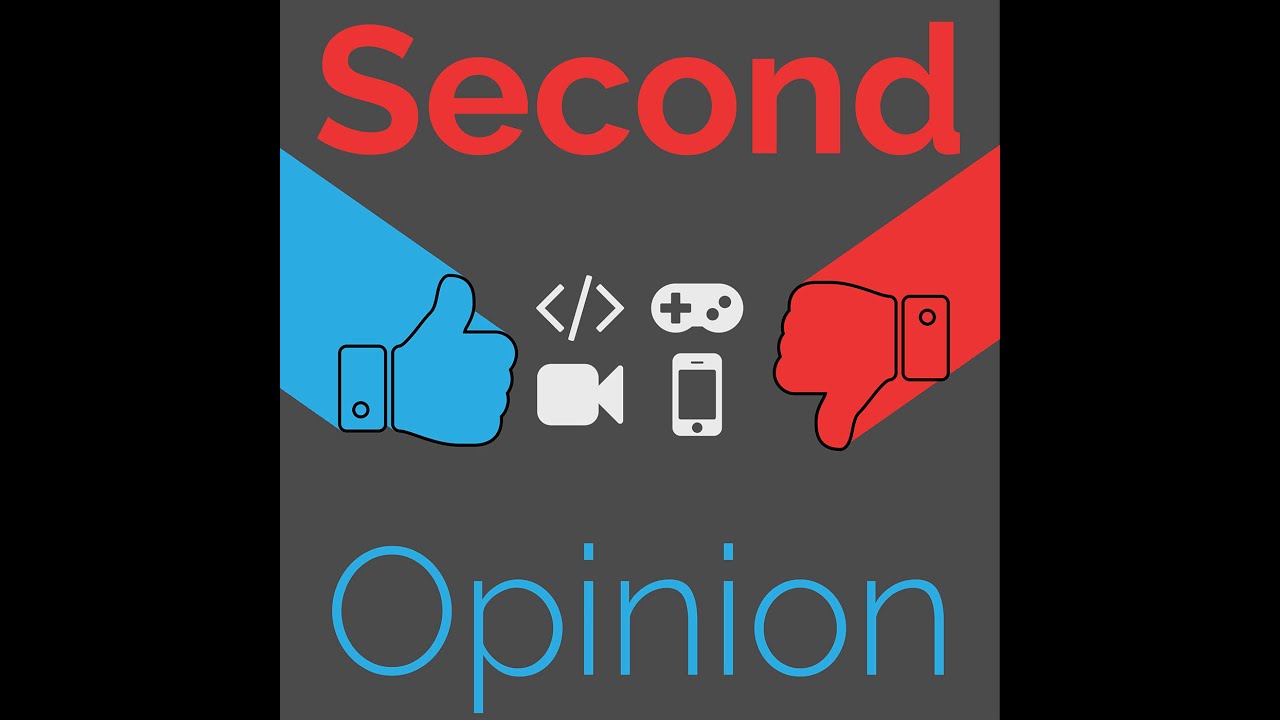The image appears to be a digital artwork or banner, possibly for a gaming or social media channel, featuring bold, contrasting colors and a simplistic design. Enclosed within thick black rectangles on both sides, the central section of the image has a neutral gray background. At the top, the word "second" appears in bold red text, while at the bottom, the word "opinion" is rendered in thin blue text. 

Prominently positioned in the middle is a blue thumbs up on the left and a red thumbs down on the right, both outlined in black with a 3D effect that gives a sense of depth. Between these opposing symbols are several white icons: a video camera on the left, flanked by a left and right arrow with a slash in the middle, a video game controller, and a cell phone on the far right. These elements combine to evoke a digital aesthetic, hinting at themes related to media, reviews, or interactive content.